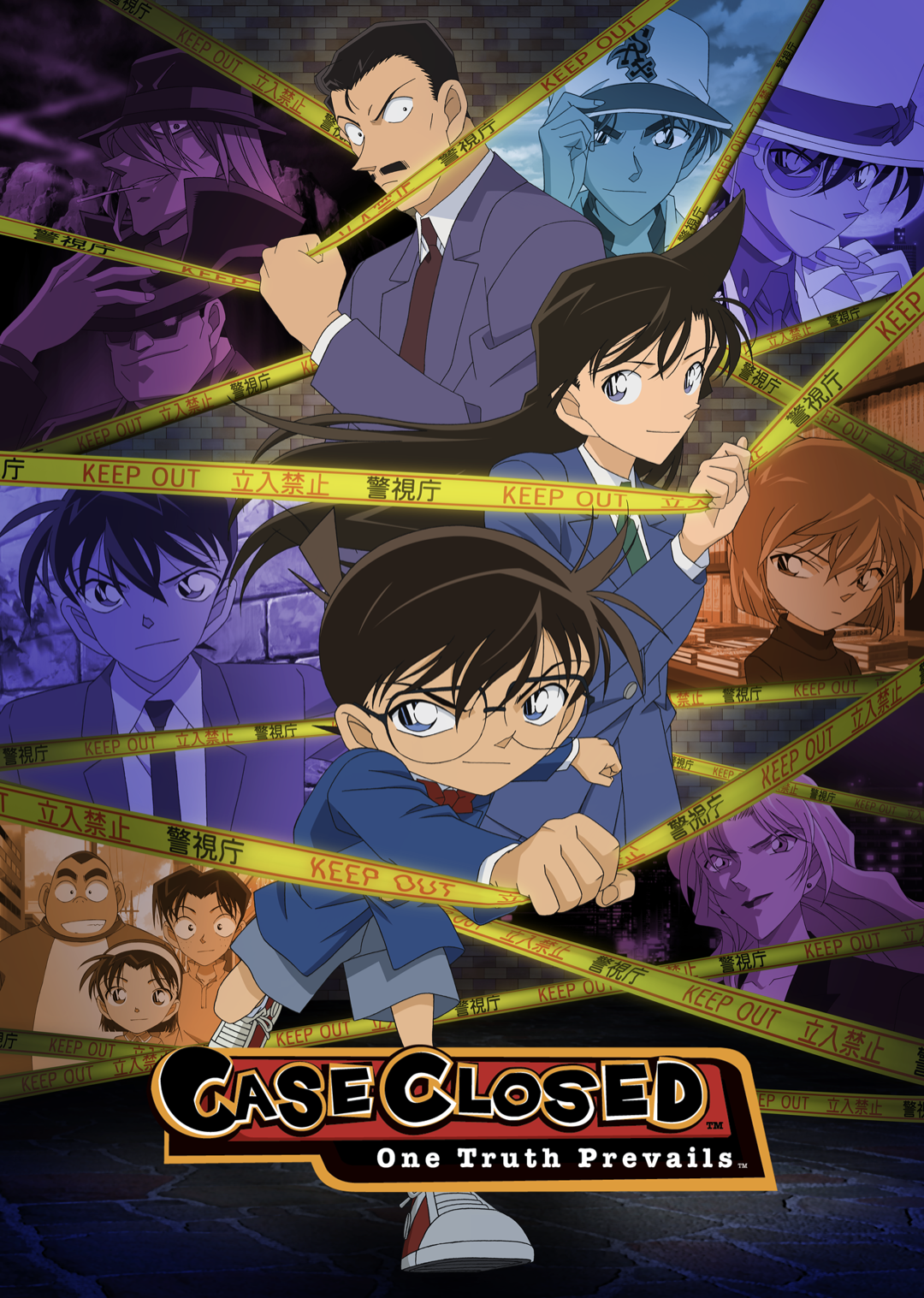This is a detailed poster for an animated series done in a distinct anime style, featuring a vibrant array of colors including blue, oxblood, grey, red, white, black, purple, orange, yellow, brown, and various shades in between. The centerpiece of the image is a kid with large blue eyes, black hair, and glasses, dressed in a blue suit jacket, red bow tie, shorts, and red sneakers. He is holding yellow ribbon tape marked "Keep out," reminiscent of a crime scene. Flanking this child are two other key characters also holding yellow ribbons: a girl in a similar blue suit and an adult man sporting a mustache in a dark purple suit. The background is a dynamic collage of smaller screenshots featuring various other characters from the series.

At the bottom of the poster is the series logo, which reads "Case Closed" in bold black capital letters with an orange outline, set against a red rectangular background with a golden border. Beneath this, in white lettering, sits the series tagline, "One truth prevails." Additional English and Chinese text is scattered throughout the image. The animated characters and vivid colors draw attention to the central theme of the series, giving the viewer a glimpse into its intriguing world.